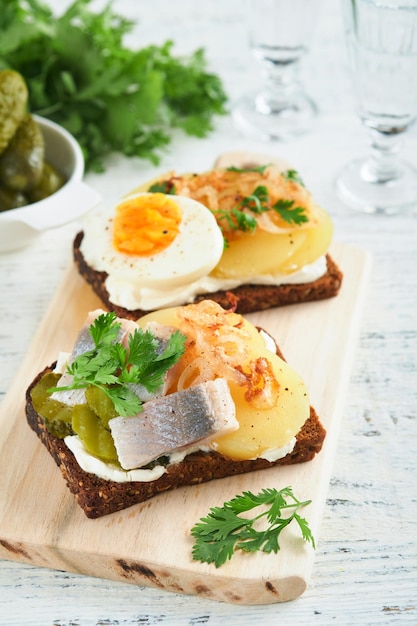The image depicts a prepared breakfast arranged on a wooden cutting board. Featured prominently are two pieces of brown toast, each topped with a delightful array of ingredients. On one piece, a generous portion of deviled eggs sits alongside pieces of salmon and garnished with what appears to be a sprinkle of fried onions and a green garnish. The other piece contains sliced fruits, possibly including pineapple, and also features half of a boiled egg. Both open-faced sandwiches are artfully presented in a bright setting that highlights the clear detail of the scene.

In the bottom right corner of the cutting board lies a piece of parsley, adding a touch of freshness to the presentation. To the left of the wooden board is a white bowl filled with pickles and a bushel of parsley. The entire arrangement rests on a surface that appears to be a gray and white dining or kitchen table. Additionally, in the top right corner of the image, there are two glass cups, contributing to the overall inviting atmosphere of the setting. The tabletop also includes a plant and what appears to be a bowl with a cactus, adding a touch of greenery to the display. The clarity and brightness of the image highlight the appetizing details of this breakfast spread.